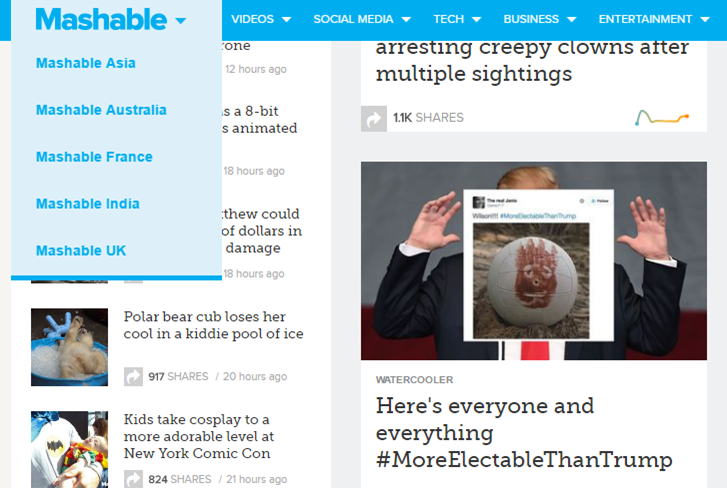This is a detailed caption describing a front page screenshot of the Mashable website:

The screenshot captures the front page of the Mashable website. Running across the top is a horizontal blue navigation bar featuring white drop-down menus and links. The leftmost menu is a large, light blue drop-down labeled "Mashable" in blue lettering. It provides options to navigate to Mashable Asia, Mashable Australia, Mashable France, Mashable India, and Mashable UK. Adjacent to it are drop-down menus for Videos, Social Media, Tech, Business, and Entertainment.

Below the navigation bar, the site is divided into two main sections. On the left side, a series of smaller articles are listed. One article's title reads, "Polar Bear Cub Loses Her Cool in a Kiddie Pool of Ice," while another is titled, "Kids Take Cosplay to a More Adorable Level at New York Comic Con."

The right side features articles with larger, eye-catching images designed to attract more readers. One prominent headline reads, "Here's Everyone and Everything Hashtag More Electable Than Trump." Above it, another article's concluding lines are visible, reading, "Arresting Creepy Clowns After Multiple Sightings." These articles feature engaging and amusing headlines aimed at drawing reader attention and providing entertainment.